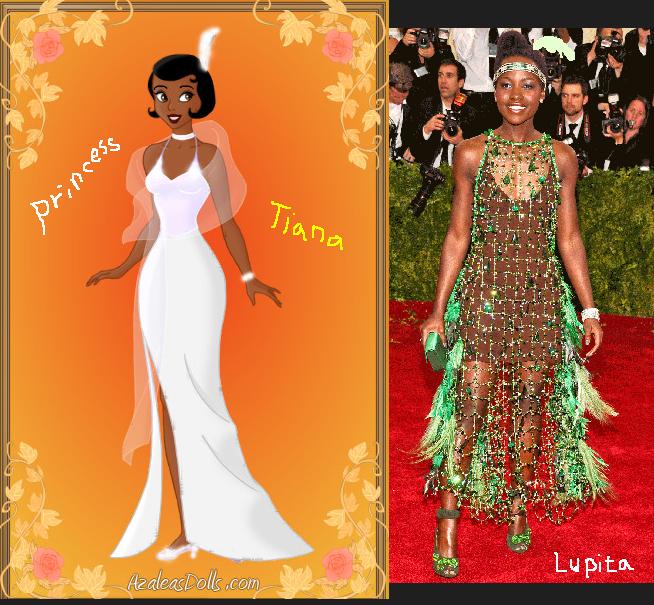The image is a composite of two separate portraits placed side-by-side, with the illustration on the left slightly larger than the photograph on the right. The illustration features an African-American woman set against an orange backdrop with a decorative gold frame featuring pink and beige floral patterns in the corners. She has short black hair, adorned with a white feather, and is smiling while looking up to her left. The woman is elegantly dressed in a long, white, strappy gown, complemented by diamond-colored high heels, a sheer wrap around her shoulders, and a white choker. Text on the illustration reads "Princess" in white on the left and "Tiana" in gold on the right, with "azaleasdolls.com" at the bottom in white script.

The photograph on the right portrays an African-American actress on a red carpet, surrounded by paparazzi and a green bush wall in the background. She is wearing a green beaded overdress paired with a dark brown mini skirt, and accessorizes with green high-heeled shoes and a matching green handbag. The photograph's text, located in the bottom right corner, reads "Lupita" in white handwritten script. Together, the images blend artistic illustration and realistic photography, creating a striking visual contrast.